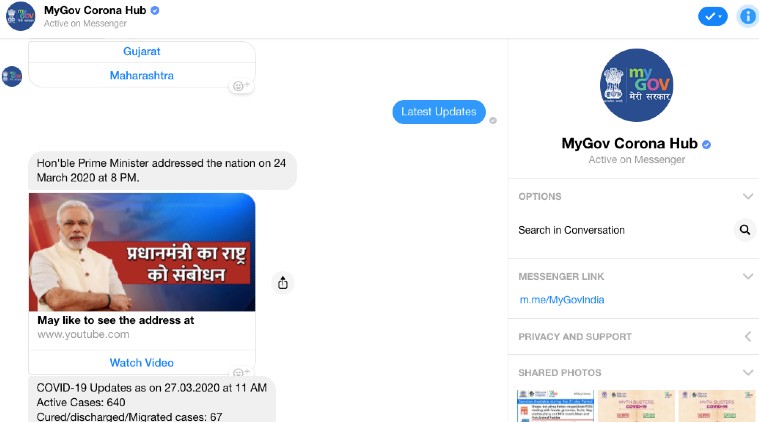This is a screenshot of a website from during the coronavirus pandemic, specifically the "MyGov Corona Hub." The top left corner of the webpage prominently displays the "MyGovCoronaHub" logo next to a blue circular icon with illegible writing inside it. Below the title, there are two clickable names in blue, which appear to be Indian names.

Further down, there's a picture of the Prime Minister of India, who is dressed in white with a white beard, facing the camera. The caption above the image reads, "Honorable Prime Minister addresses the nation on 24 March 2020 at 8 p.m." The image suggests that the Prime Minister's address can be viewed as a YouTube video, with a clickable option beneath the picture to watch it.

Below the video, there is an update on COVID-19 statistics as of March 27, 2020, at 11 a.m. The stats indicate there are 640 active cases and 67 discharged or migrated cases.

To the right of this content, there appears to be a sidebar labeled "MyCoronaHub," which provides options for users such as search and conversation. There are also links for Messenger, further information, privacy and support, and shared photos, all written in blue for easy access.